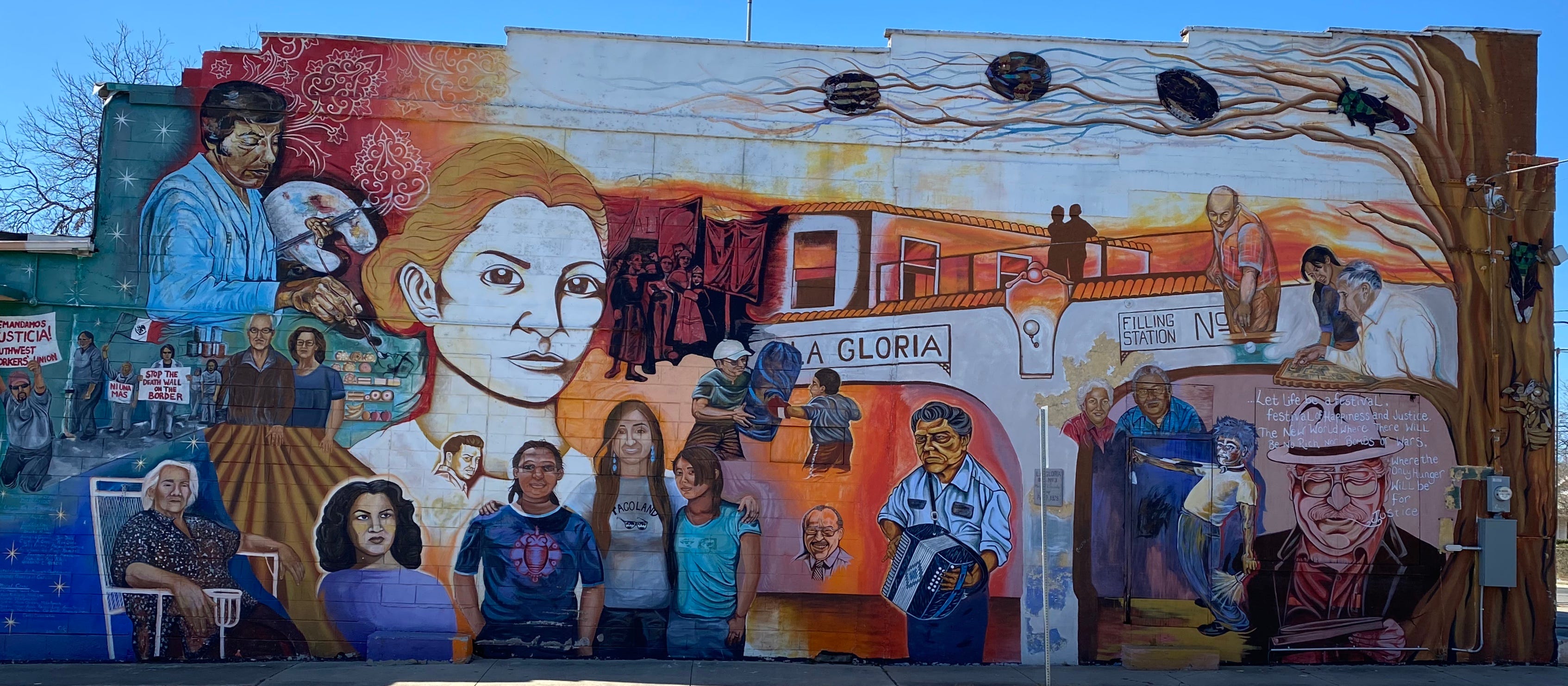This vibrant mural, set against a clear daytime sky on the side of a building, is a rich tapestry of various scenes and characters. To the left, a painter is captured mid-action, holding his paintboard and brushes, seemingly painting the very mural he is a part of. Below him, a diverse group of smaller figures protest for justice, with signs in hand and what appears to be the Mexican flag included in the artwork. Adjacent to this, an elderly Mexican grandmother sits in a chair, observing the scene around her. Towards the center, a medium-aged group gathers around a table, while a large, dignified woman stands as a prominent figure, surrounded by various individuals. Further to the left, a painted building that resembles a cantina or gas station emerges, featuring a musician joyfully playing the accordion and children engaging in a playful boxing match. On the right side of the mural, a towering tree painted up the side of the building intertwines with the scene, its branches adorned with black objects and possibly animals. The intricate details, from a 1960s-style police officer to families and people from all walks of life, bring this mural to life, showcasing a rich tapestry of culture, community, and activism.